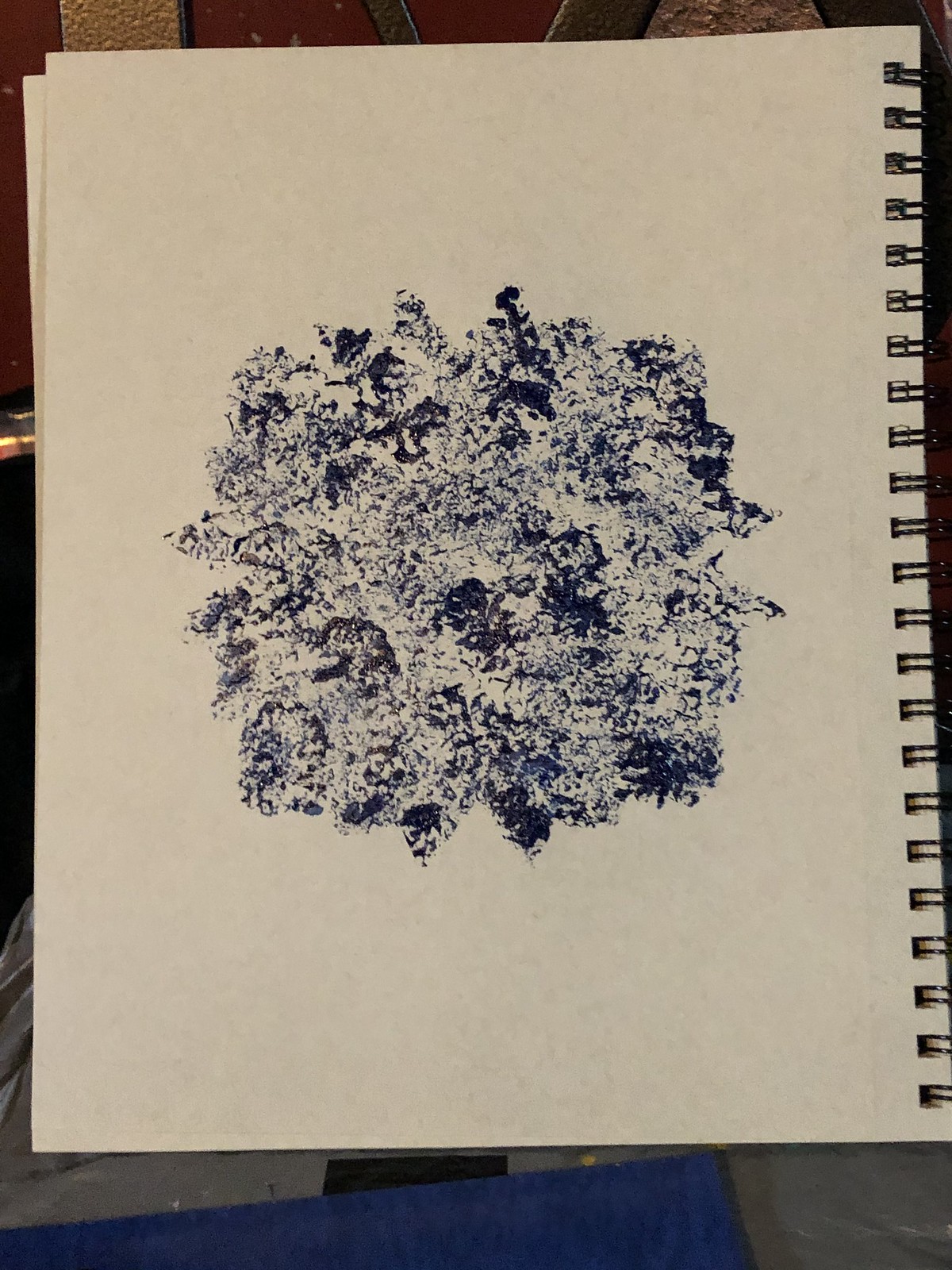This image features a detailed sketch on a sheet of pristine white drawing paper, which is set within a binder. The paper is turned to a single page, with the sketch itself depicting what appears to be a sprawling, dense bush. The bush is rendered in dark tones, possibly black or very dark blue, which contrasts vividly against the white background of the page.

In the background, faintly visible, are objects that resemble wooden structures, likely forming a wall. These elements provide a subtle backdrop to the forefront sketch. The binder seems to be positioned upright or possibly leaning against a surface for support.

Beneath the binder, there is a fabric with a texture and color similar to blue jeans, adding a coarse, casual feel to the setting. The edges of the binder's foliage design are outlined in black, highlighting the openings of the drawing paper and contributing to the overall frame of the artwork.